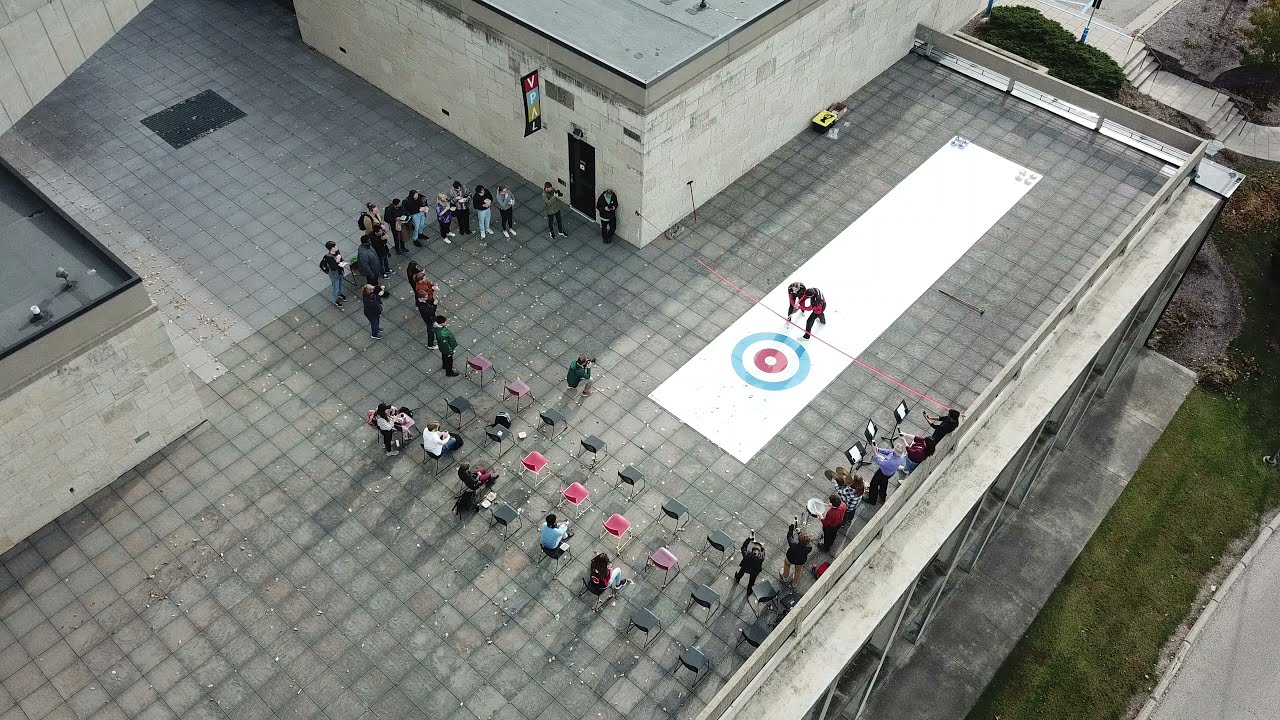This is an aerial photograph taken during the daytime, likely from a drone, capturing the top of a two-story building, which could be an office building or perhaps a library. The roof, covered in gray cinder blocks or concrete, is the central focus of the image where some organized activity is taking place. 

In the upper right-hand section of the roof, a long white rectangular mat has been laid out. At the far end of this mat is a target with four concentric circles colored white, red, white, and blue, resembling a bullseye. A thin red ribbon stretches across the mat, dividing the target area from the main area of activity, which includes two individuals. These people, dressed in red and black uniforms, appear to be engaged in an athletic competition, possibly curling or wrestling.

Various observers surround the mat; some are seated in chairs set up towards one end of the white rectangle, while others stand, some taking notes or recording the event. The roof also features a band playing music near the right-hand ledge, adding to the lively atmosphere. A doorway leading to the lower floors of the building is visible, and a banner with the letters "VPAL," whose meaning is unclear, is prominently displayed.

This clear and sunny day highlights the details and makes the rooftop event stand out against the urban backdrop.